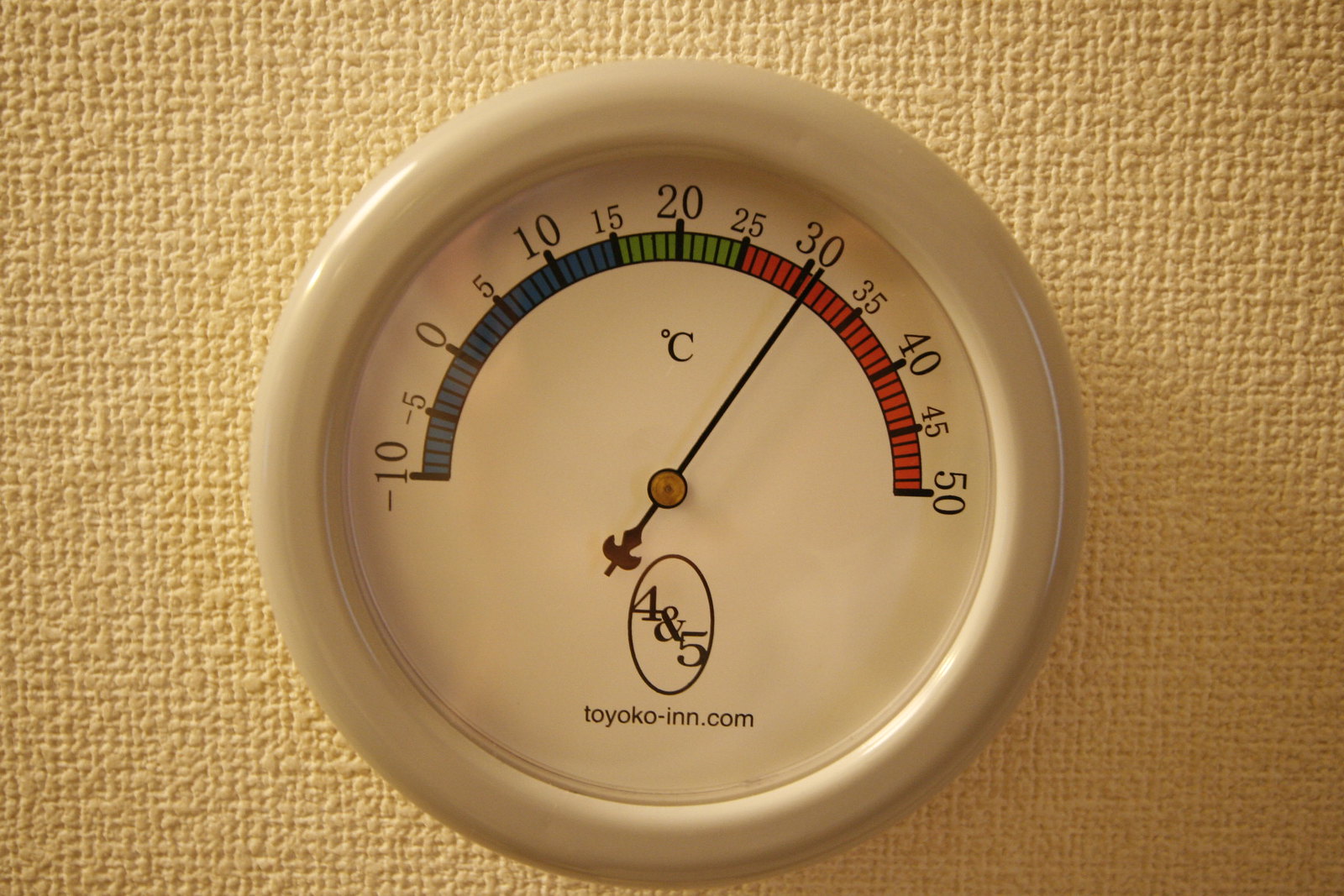This photograph showcases an antique-style, round wall thermometer with a clock-face design, mounted on a yellow, matte-textured wall. The thermometer's casing is made of white plastic, complementing its white interface. At the bottom, the device features the website "toyokoinn.com." Just above the website, there is a vertically oriented oval logo containing the numbers "4" and "5." The thermometer's gauge ranges from -10 to 50 degrees Celsius, segmented by color: blue from -10 to 15 degrees, green from 15 to 25 degrees, and red from 25 to 50 degrees. The central dial prominently displays the unit "°C" for Celsius, with the needle indicating a temperature of approximately 31°C.